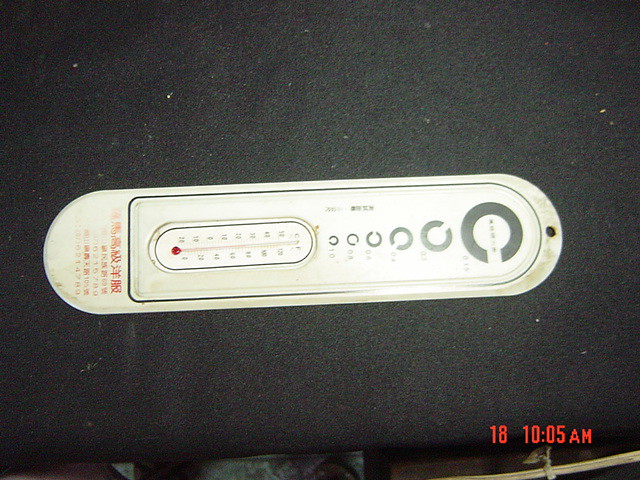The photograph showcases a dingy white thermometer, which appears to be made of plastic or thin metal, lying horizontally on a black surface. The thermometer, which has the form factor of one typically meant to be nailed to a wall, features a series of circular gauges with notches at its top. These printed circles contain illegible markings that seem to be in Chinese, suggesting foreign manufacture. Part of an advertising giveaway, the thermometer has a smaller thermometer embedded at its base. Additionally, there is more text, also in what appears to be Chinese or Korean, located beneath the thermometer. The timestamp "18 10 05 AM" in red digital font is prominently displayed at the bottom right corner of the image, adding a sense of captured moment to the otherwise utilitarian scene.